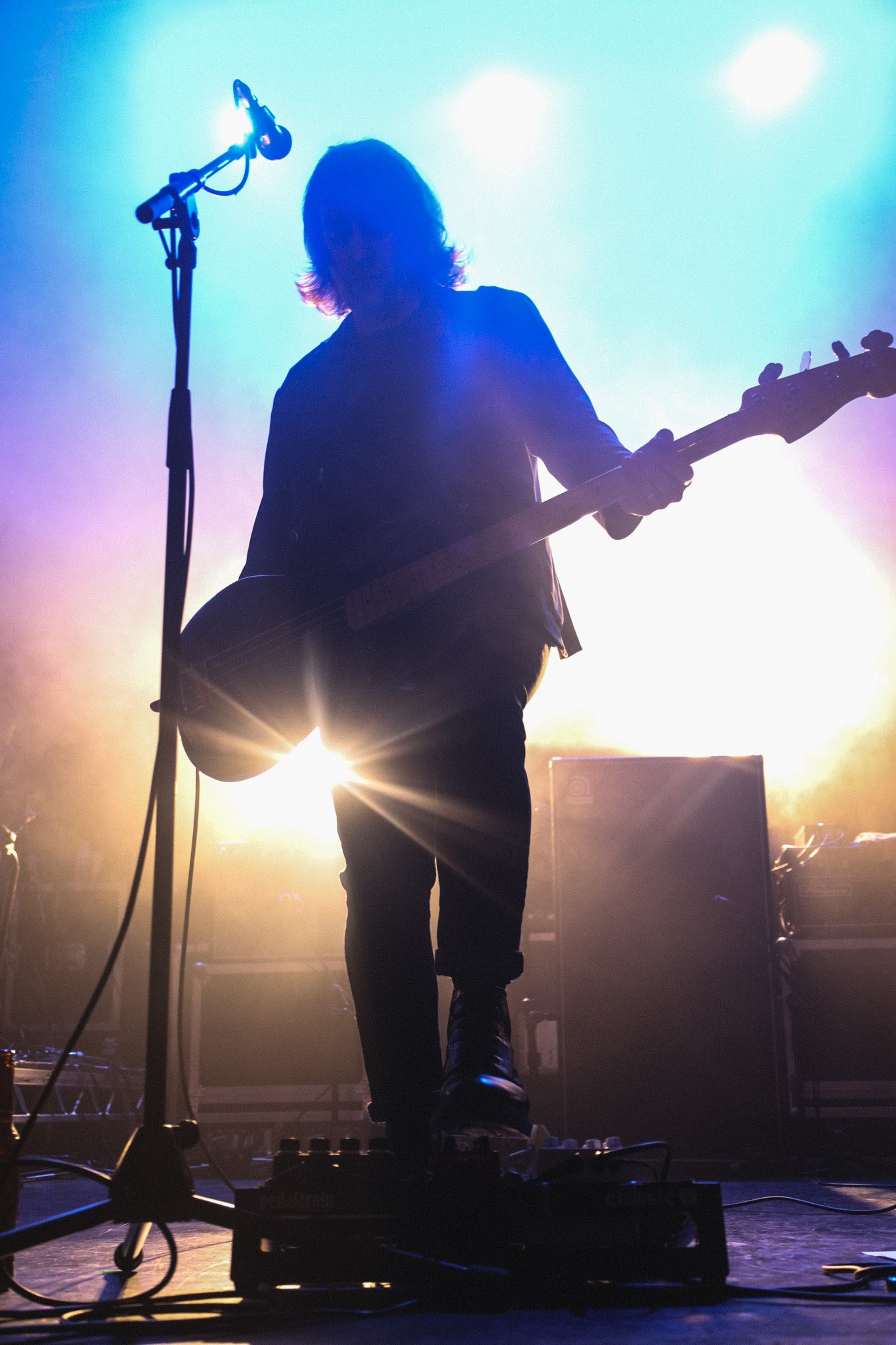The image depicts a silhouetted man, likely a guitar player, standing on a stage against a backdrop of a bright sky with the sun shining intensely. His face and detailed features are obscured by the stark contrast between his darkened outline and the bright light behind him. He has shoulder-length hair, wears boots and dark pants, and dons a long-sleeved shirt. One of his arms is positioned with his hand on the guitar, while the other arm is partially hidden behind the instrument. His guitar, which he holds across his body, features a rounded wooden base with strings and a V-shaped headstock. To his left, a microphone stands on a pole, and below him, his foot is engaged with some form of control box equipment on the ground. Surrounding him are large black rectangular speakers, amplifying his music. The stage itself is gray, with hues of yellow, blue, and purple spotlights in the background, enhancing the ethereal atmosphere of the performance.